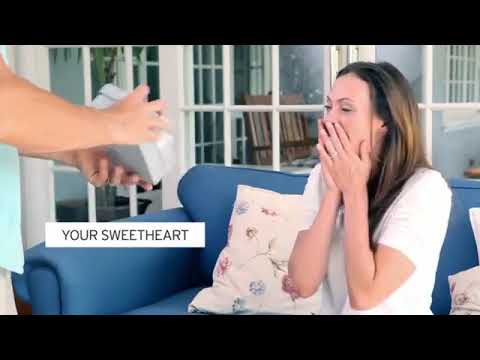The image shows a woman with long, straight brown hair sitting on a blue sofa adorned with white floral pillows. She wears a white t-shirt and appears to be excited or surprised, covering her mouth with both hands, her arms bent at the elbows. A man, partially visible, extends a small square white gift box towards her, his aquamarine shirted forearms being the only parts of him visible as he stands off to the left side of the frame. The background features a glass-paned door or window with white grid-like panes, suggesting an outdoor patio setting. The picture is framed with thick black horizontal borders at the top and bottom, and in the lower left corner, a small white rectangle contains the text "YOUR SWEETHEART" in blue, all capital letters.